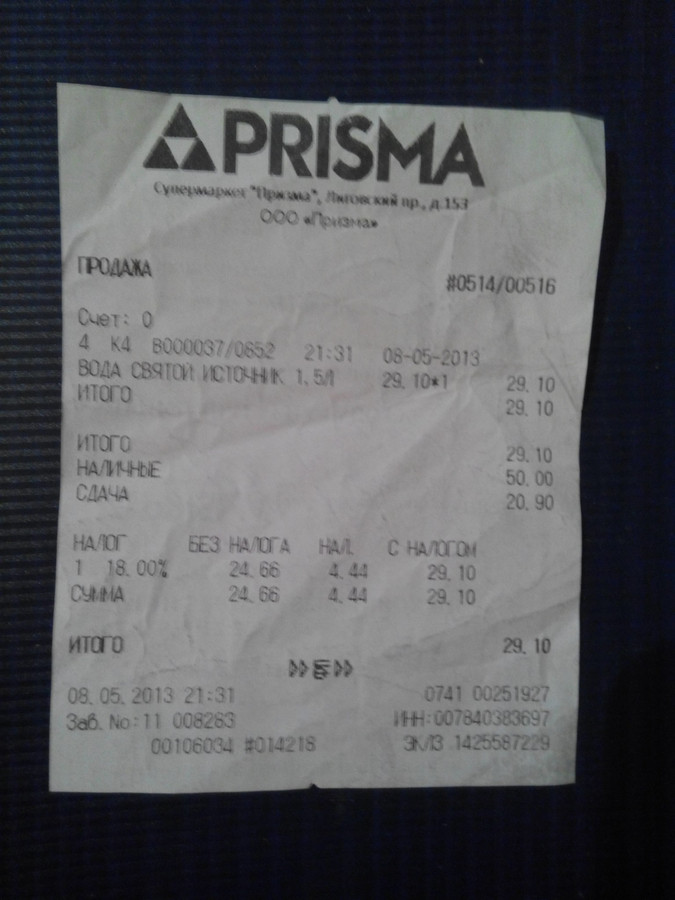This image displays a close-up photograph of a white receipt with black text, set against a black and gray herringbone or tweed background. At the top of the receipt, the logo "Prisma" is prominently displayed in large black letters, accompanied by a distinctive triangular logo featuring a black triangle with an upside-down white triangle inside it. Below the logo, the text is mostly illegible, appearing to be either in a foreign language or written in abbreviated form, making it difficult to ascertain the specific items purchased. The receipt includes numerous listed items amounting to a total of $29.10. Additional numbers are visible beneath this total, including another instance of $29.10, as well as $50 and $20.90, although their contextual significance is unclear. The date on the receipt reads 8-05-2013, indicating either August 5th or May 8th of 2013. Additionally, there is a mention of "18%", which could potentially refer to a tax or tip.